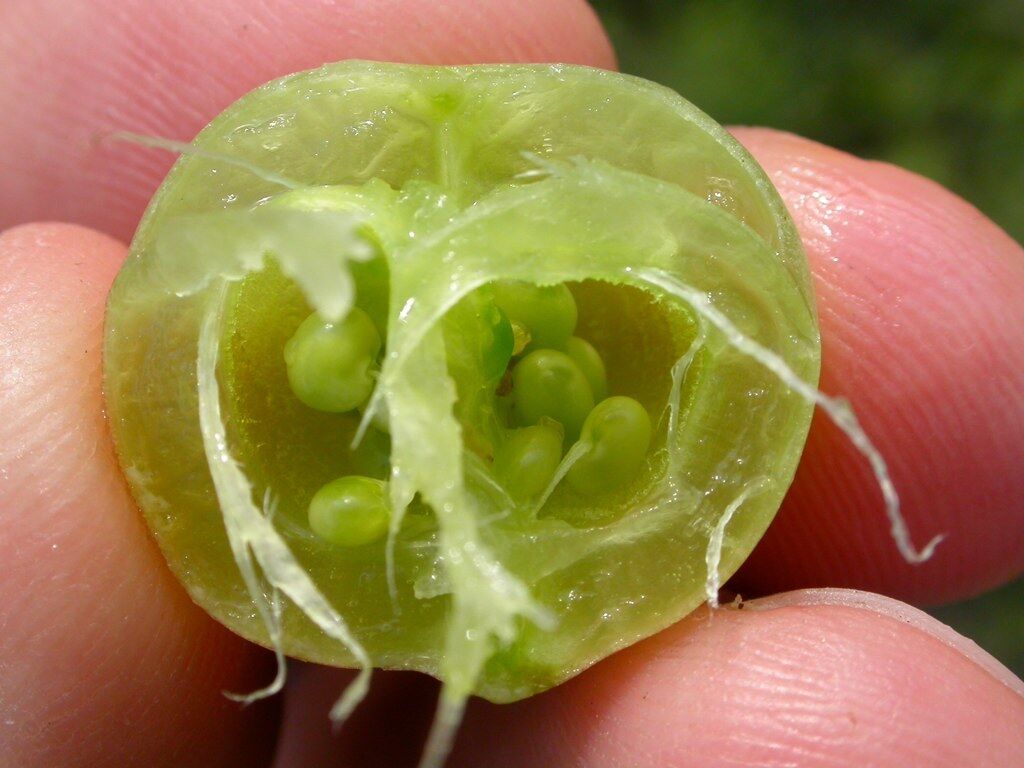This extreme close-up colored photo captures a cross-section of a small, fleshy fruit, likely a green grape, nestled in someone's hand. The size of the fruit is just slightly larger than the width of a finger. Its light green, nearly transparent flesh reveals a number of very small seeds inside. The fruit is being held delicately by four fingers, and despite the prominent black background in the upper right of the frame, the focus remains sharply on the hand and the fruit. The fruit’s shiny, almost plastic-like appearance gives it an intriguing gloss, making it look as though it could be artificial. The mysterious, punctured hole within the fruit further reveals clusters of tiny seeds, adding to the detailed textural complexity of the image.